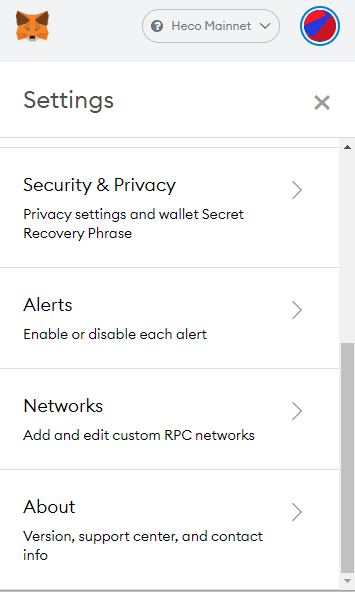The image is a screenshot apparently taken from a mobile phone. At the top of the screenshot, there is a gray rectangular bar. In the top-left corner of this gray bar, there is an icon depicting a stylized red fox head, rendered in a cartoonish style and looking straight ahead. To the right of this icon, there is an outline of an oval. In the center of this oval is a black circle featuring a gray question mark. Adjacent to this, the text "HEKOMENE" is displayed in black font. Following this, there is a downward-pointing arrow. Next to this, on the far right, is a blue circle enclosing a red circle with a blue slash running through it.

Beneath this top section, the background of the page is white. In the top-left corner, the word "SETTINGS" is prominently displayed in large black font. In the top-right corner of this white section, there is a gray "X" icon. Below these elements, two vertical black lines are visible. Further down, the text "SECURITY & PRIVACY" is displayed in black font, followed by "PRIVACY SETTINGS & WALLET SECRET RECOVERY PHRASE." To the right of this text, there is a right-pointing arrow. A black horizontal line separates this section from the one below.

The next section features the text "ALERTS" in black font, followed by the phrase "ENABLE OR DISABLE EACH ALERT," with a right-pointing arrow to the right of the text. Another black horizontal line separates this section from the final one.

The bottom section of the page displays the text "NETWORKS" in black font, followed by the phrase "ADD ONE & EDIT CUSTOM RPC NETWORKS." This text is also accompanied by a right-pointing arrow on its right side.